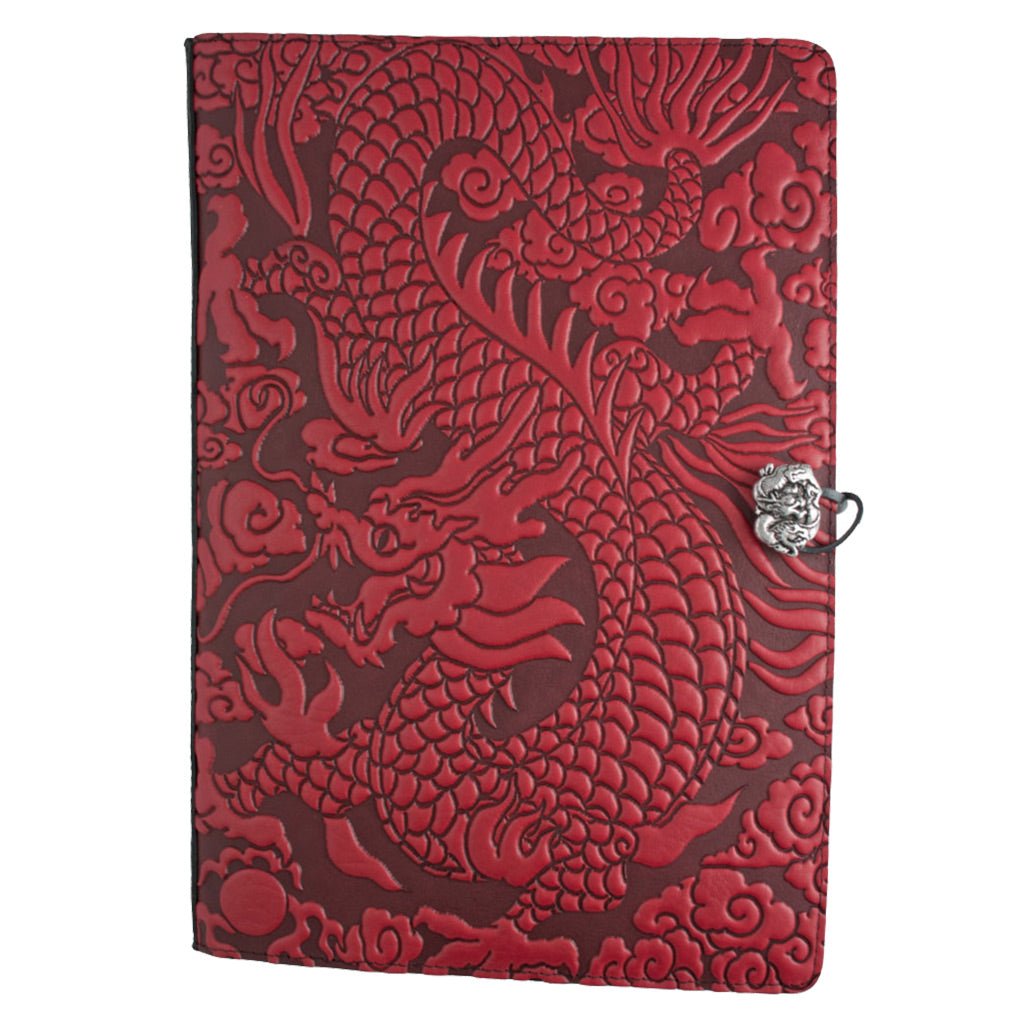This angled photograph captures the intricate cover of a leather notebook or diary, adorned with elaborate designs. The cover is crafted in rich red leather, embossed with a detailed image of a Chinese dragon. The dragon, characterized by rough scales and a tail reminiscent of a fish, wraps majestically around the entire cover. Its head is oriented to the left, with its body interwoven with a background teeming with fanciful swirls and floral motifs, imparting a sense of ornate intricacy. Notably, a small, ornate silver clasp, shaped like a dragon, is positioned at the right center, accompanied by a black string-like clasp that secures the book. The overall design is accentuated by etched patterns and raised textures, giving the impression of an artfully carved masterpiece.